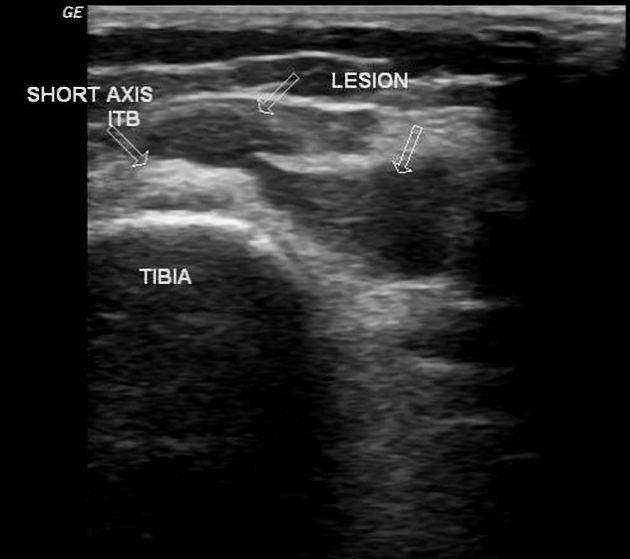The black-and-white medical image, likely an X-ray or possibly an ultrasound, showcases the pelvis region in a zoomed-in and blurry fashion, hinting at its hospital origin. Key anatomical features are marked with arrows: the tibia is labeled, alongside regions with lesions identified in two parts of the pelvis. Additionally, the short axis and ITB are noted within the image. The overall appearance is fuzzy, implying it could be an ultrasound. On the left side of the photograph, a black strip is visible, bearing the label "GE" at the top, indicating the equipment brand. The image concentrates on a single leg, presenting a detailed view of potential patient issues post-injury.